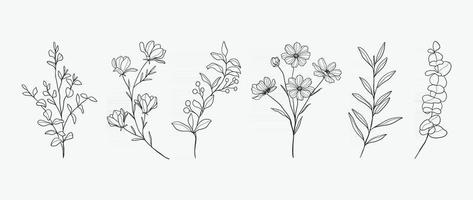This black-and-white, hand-drawn image on a white background features six meticulously detailed flower branches, each showcasing a unique botanical specimen. The first branch displays opposing ovate leaves, symmetrically arranged along the stem. The second branch is crowned with four butterflies-like blossoms, their narrow, lanciate leaves giving the impression of delicate movement. The third drawing exhibits broad, laurel-like leaves accompanied by clusters of round berries, reminiscent of ivy. The fourth sketch captures the intricate beauty of daisies, so finely detailed that one can almost perceive the yellow hue through the monochrome. The fifth illustration is a sparse sprig of fern with elongated, slender leaves. The final branch, on the far right, shows what appear to be large, fluffy cotton bolls grouped closely together, resembling marshmallows on a stick. Each detailed pencil drawing highlights the distinct characteristics of the flowers and plants, making the collection a study in botanical artistry.